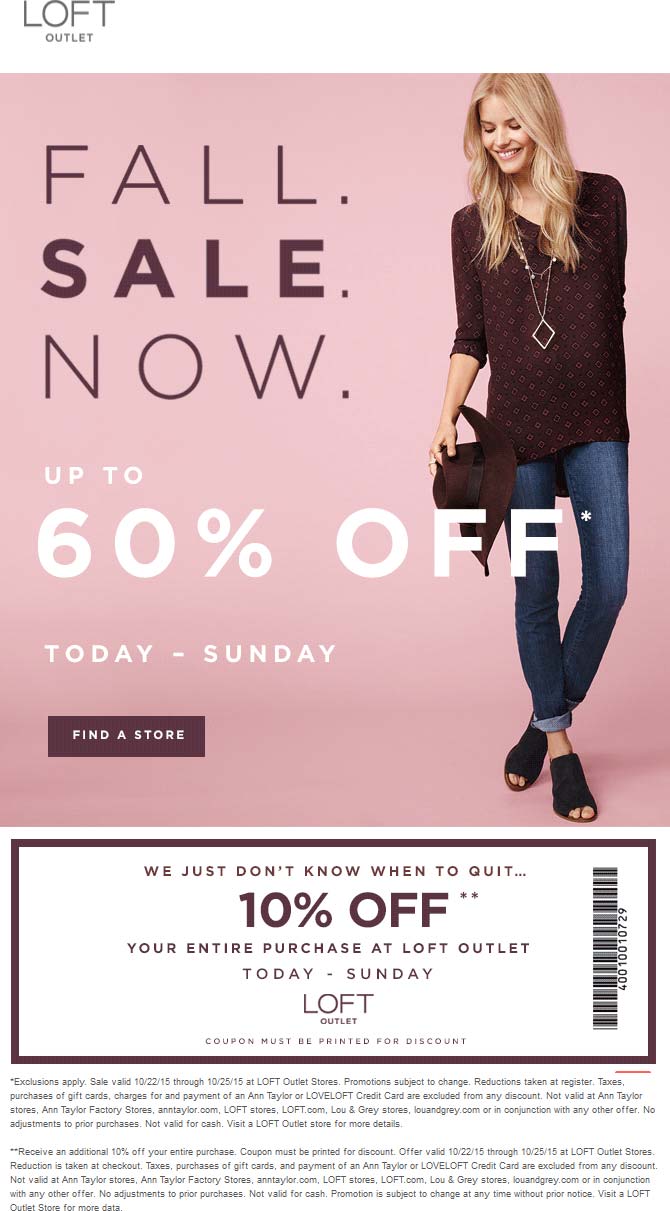The image features a vibrant promotional banner for Loft Outlet, prominently displayed at the top in bold purple letters. Below, a striking purple box announces a "Fall Sale Now," offering discounts of up to 60% off, valid from today through Sunday. Adjacent to this is a sleek black button labeled "Find a Store."

Centrally featured is a stylish image of a blonde-haired woman wearing a chic black sweater paired with blue jeans, accessorized with a black purse and a gleaming gold necklace. The image is complemented by a prominent text overlay reading, "We just don't know when to quit," emphasizing an additional 10% off your entire purchase at Loft Outlet within the same sale period.

The promotional material also includes an image of the coupon with a black outline, featuring a unique barcode to redeem the discount. Beneath the coupon, detailed terms and conditions are provided for clarity. This enticing promotion combines the allure of a generous 60% off with an added 10% savings, encouraging customers to visit Loft Outlet.